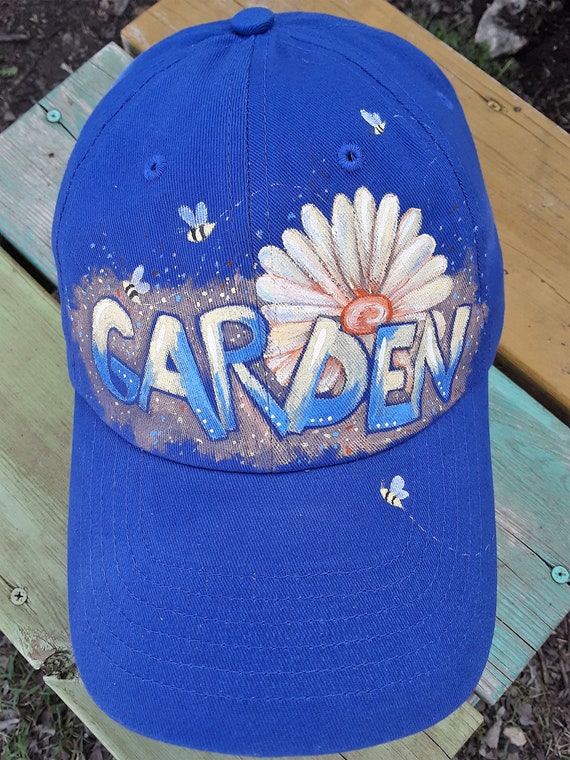This image features a detailed, homemade royal blue baseball cap adorned with whimsical designs. The cap prominently displays the word "GARDEN" across the front, with letters that are creatively styled with a gradient effect—blue on the lower part and creamy yellow on the upper part. Surrounding the text and adding to the cap's charm is a large, vibrant flower, featuring white petals and an orange center, covering much of the right side of the cap just above the brim. Scattered around the word "GARDEN" are small, playful bees, with four in total—three on the cap's main body and one on the brim—each accompanied by delicate flight lines. The cap is positioned atop three pieces of plywood nailed together, possibly forming a crude stand or crate. The scene's background includes scattered leaves, grass, dirt, and small rocks, which subtly frame the central focus on the intricately decorated ball cap. The craftsmanship involved in creating this cap suggests it’s a charming, handmade project, rather than a commercially purchased item.